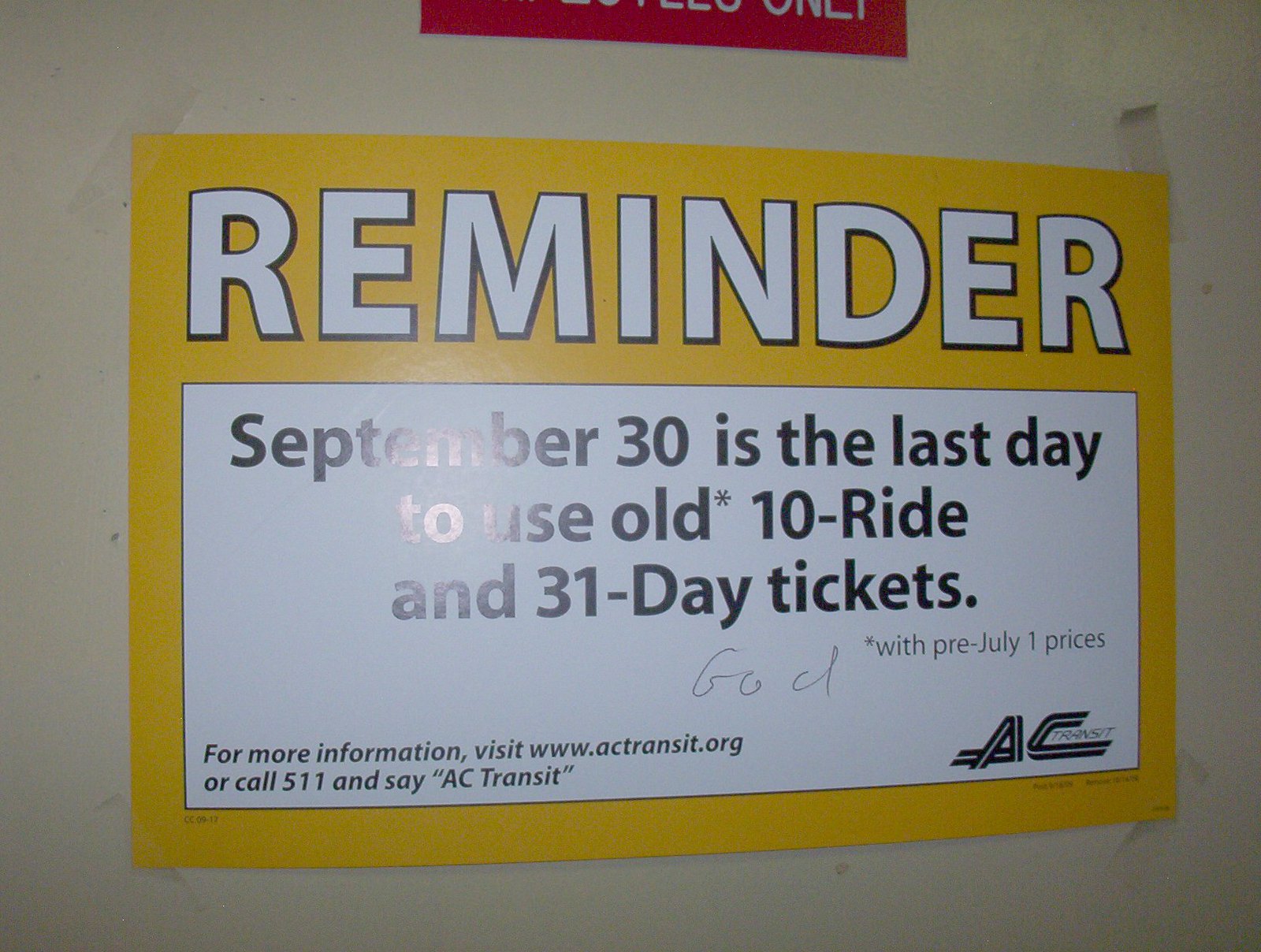The photograph captures a notice posted on a white wall. Centrally positioned, the main sign features a prominent yellow border, thinner on the bottom and sides and wider on top, with the header "REMINDER" in large white capital letters. Below this, printed on a white rectangular section, the black text reads: "September 30 is the last day to use old 10-day and 31-day tickets with pre-July 1st prices." An asterisk (*) marks the statement. In the bottom left corner, directives for more information are provided, stating "visit www.actransit.org or call 511 and say AC Transit." The bottom right corner bears the AC Transit logo, characterized by stylized letters "A" and "C" forming street-like graphics with "TRANSIT" inscribed in the "C." Above the main sign, a partially visible red sign with white text appears to read "EMPLOYEES ONLY." Additionally, the main sign has graffiti with the word "GOD" written in ink.